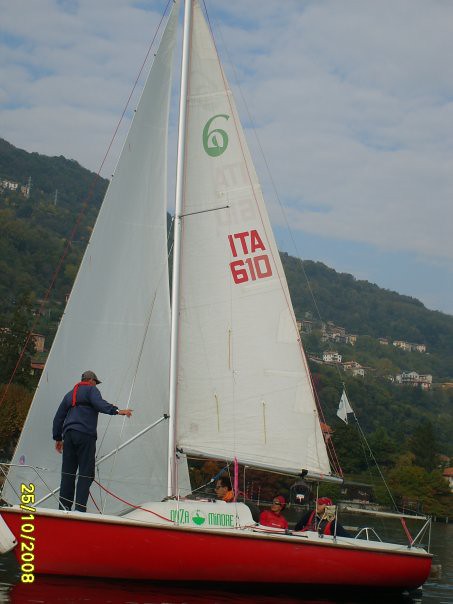The photograph, rectangular in shape and of mediocre quality, appears to be taken with an older-style camera, as evidenced by the yellow date stamp reading "25-10-2008" in the lower left corner. The central focus of the image is a small sailboat, approximately 10 to 15 feet in length, with a red hull and white sails. The sail is marked with a green logo resembling the number six near the top and the text "ITA 610" in red beneath it. The boat is sailing on a calm body of water, with a man standing at the front, manning the sails. He is clad in a blue jacket, red scarf, green baseball cap, and dark pants. Three other individuals are seated towards the back of the boat. In the backdrop, there's a wooded hillside, densely populated with trees and scattered houses. The sky is light blue, accented with numerous white clouds, suggesting a sunny yet partially cloudy day.